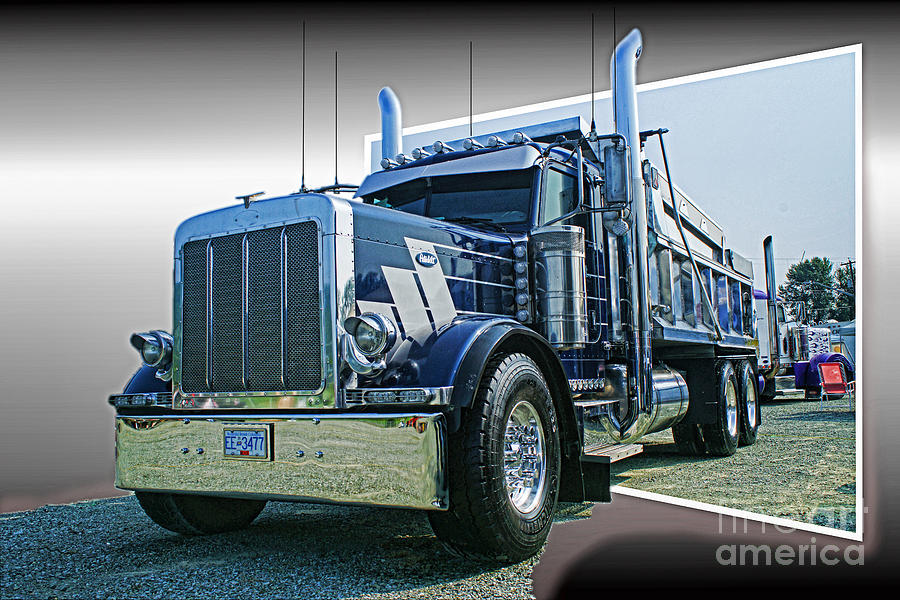This is a highly detailed, full-color artistic piece that features an intricate depiction of a large blue Peterbilt dump truck in pristine condition. The truck is showcased in a horizontal rectangular image, appearing to drive out of a Polaroid-style photograph, creating an optical illusion. The truck's chrome features, such as the grill, front bumper, lights housing, gas tank, and exhaust pipes, shine brilliantly against the dark blue, perfectly maintained paintwork of the truck and truck bed. The illusion shows the truck protruding out to the left of the skewed picture frame, with gravel visible beneath it in the bottom left corner. The background within the frame consists of a white gradient fading into black at the top and bottom, giving way to a grassy field and another semi-truck in the distance. Surrounding the image, there is no discernible border or specific background, enhancing the optical illusion effect. A watermark reading "Fine Art America" is positioned in the lower right-hand corner of the image. Color elements in the scene include metallic silver, black, blue, red, yellow, and green, adding to the vividness and realism of the artwork.